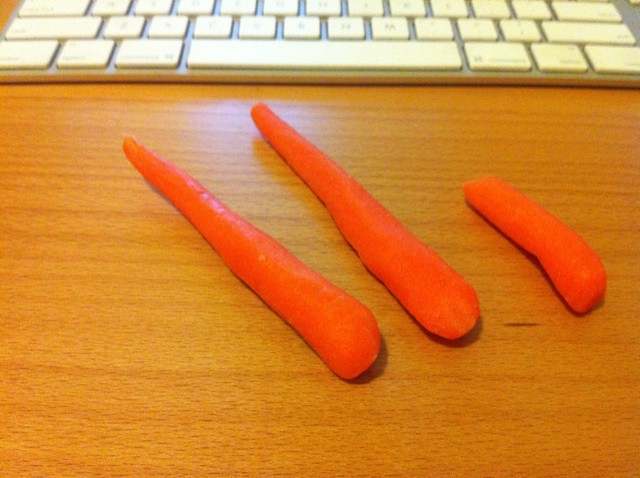The photograph showcases a trio of peeled carrots placed diagonally on a light and dark brown wooden table with a visible grain pattern. The tips of the carrots point towards the upper left corner of the image. The two larger carrots on the left are approximately the same length, around 10 inches, while the smaller, irregularly-shaped carrot on the right is about half their size. Some irregularities on the smaller carrot suggest it might have been partially eaten or chopped. The vibrant red-orange color of the carrots is accentuated by a blend of natural and artificial lighting, giving them a fluorescent, almost hot lava appearance with reflections visible on their surfaces. In the background, there is a thin, white computer keyboard, partially cropped out, revealing just the first two and a half rows of keys. The keyboard sits atop the table and provides a stark contrast to the vivid brightness of the carrots.